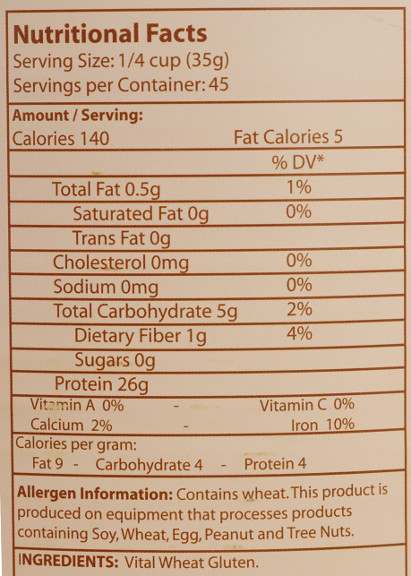This photograph features a detailed close-up of a substantial, rectangular Nutrition Facts panel prominently displayed on a pinkish background. The panel is surrounded by a burgundy border, matching its burgundy text and headings. At the top, the panel clearly states "Nutritional Facts," followed by crucial information such as "Serving size: 1/4 cup" and "Servings per container: 45." Toward the bottom of the panel, there is a section dedicated to allergen information. The very bottom of the image hints at an ingredients list, although it is partially cut off and not fully visible in the frame. The entire image is a tall, zoomed-in shot that solely focuses on the Nutrition Facts, leaving the associated product unidentified.